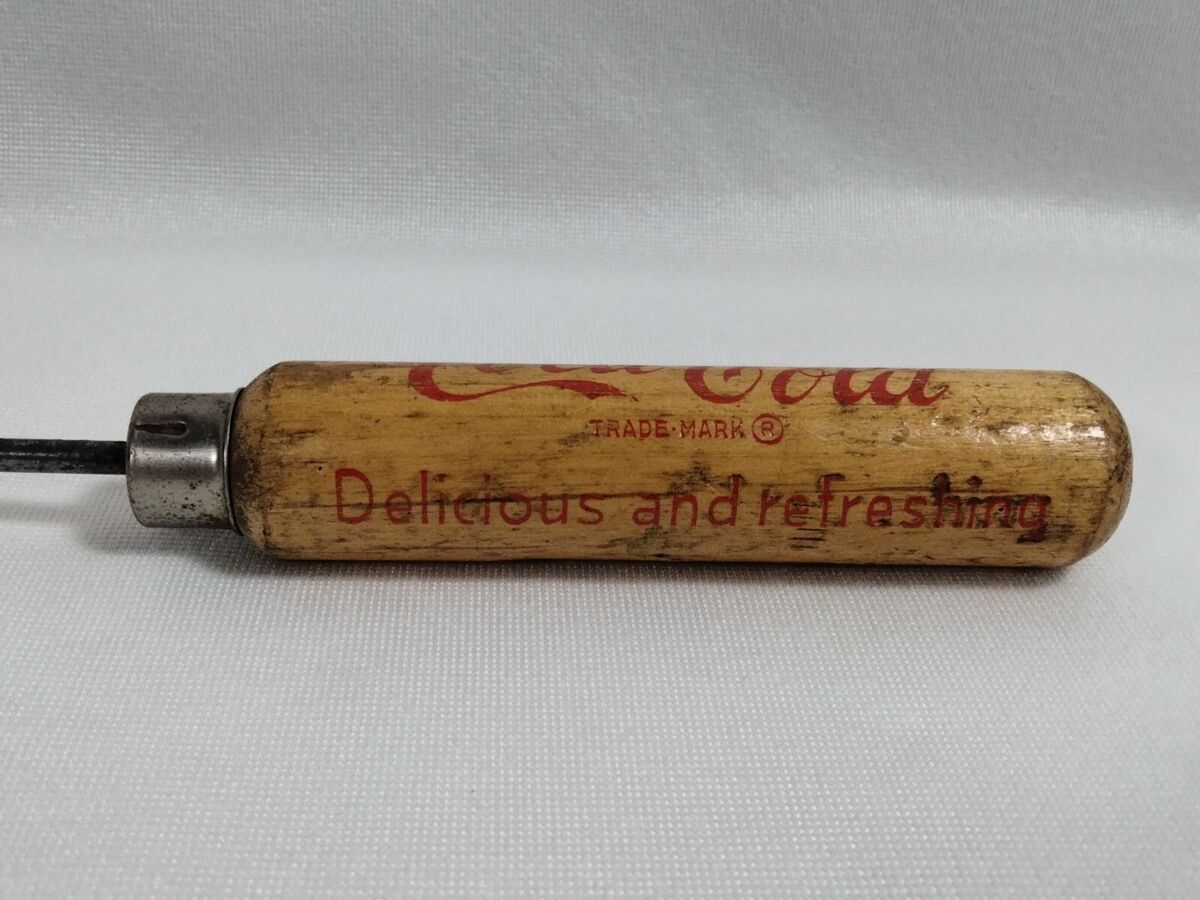The image features a vintage wooden tool that resembles a rolling pin or a baseball bat, made from light gray wood. The tool's wooden surface displays the iconic Coca-Cola branding with the text "Coca-Cola Trademark" followed by "Delicious and Refreshing", both inscribed in red. A piece of metal is affixed to the left end of the tool, from which a smaller metal rod protrudes. The entire object appears weathered, with visible scuff marks and chips, and it seems to be lacquered or coated with a shiny finish. This item is set against a white background that has a woven texture, possibly cotton, suggesting it might be displayed like a museum piece. The lighting in the image is even, and there are reflective highlights on both the metal and wooden parts of the tool. This well-preserved, historic artifact clearly ties into Coca-Cola's rich heritage.